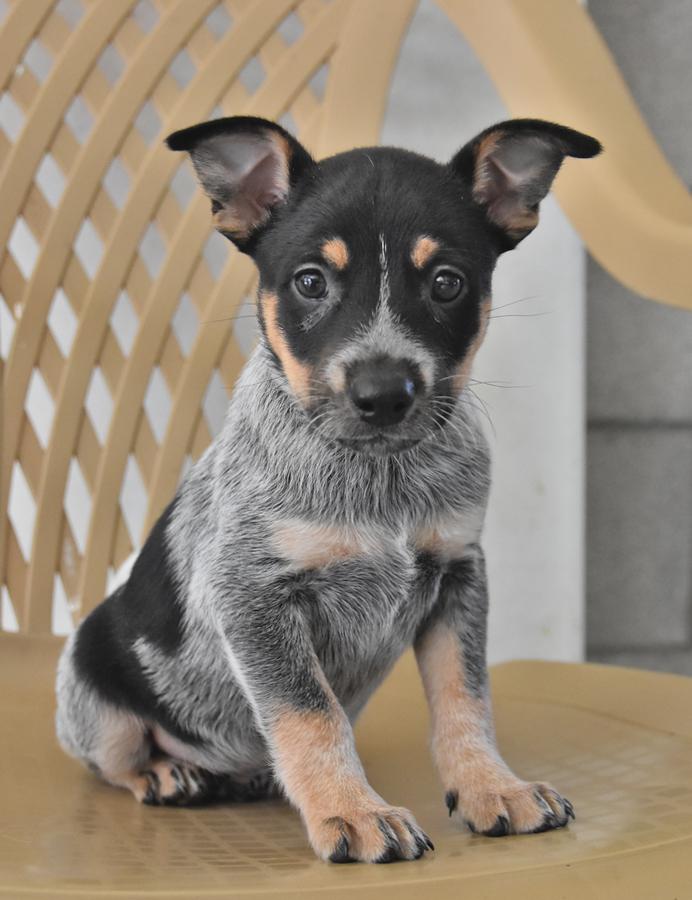This indoor photograph captures a small, mixed-breed puppy sitting on a brown plastic chair, featuring slats curving left and right. The portrait showcases the entire dog's body, making the rectangular image approximately six inches high and four inches wide. The puppy, resembling a heeler mix with some Rottweiler-like markings, is attentively looking directly at the camera with perked-up ears. Its predominantly black head is accented with small brown eyebrows, tan cheek lines, and a thin gray stripe down the snout leading to its black nose. Inside the ears, you see tufts of brown, along with hints of gray and pink. The pup's legs exhibit a light gray color with black undertones, transitioning to brown fur and ending with black nails. Its chest displays a distinct brown band beneath a patch of white, while its back has darker black patches amidst predominantly gray fur, particularly along the belly and toward the rear. The chair's brown plastic material complements the puppy's coat, creating a warm and homely atmosphere in the photo.